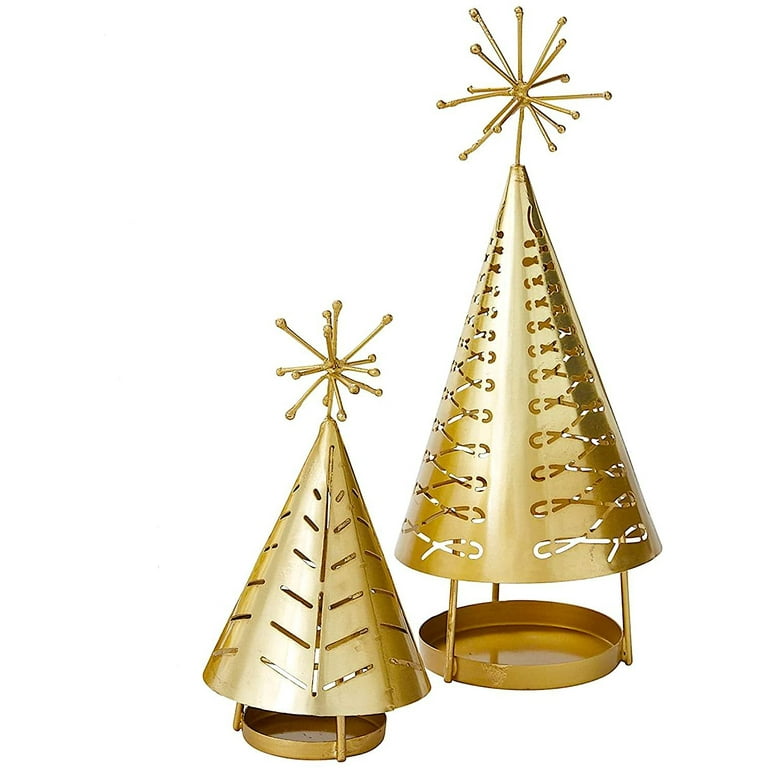This is a sales picture of two gold, stylized Christmas tree tea light candle holders, displayed on a white background. The holders feature circular bases with short lips, creating a platform suitable for placing candles. Each tree-shaped cone is held up by three metal posts. The smaller tree, positioned on the left, has vertical line slits cut through its surface, while the larger tree on the right showcases a crisscross pattern. Both trees are topped with a 3D star-like figure, featuring a central point surrounded by smaller points, each ending in a tiny circle. The golden brass color and intricate cutouts allow for candlelight to shine through, enhancing the decorative appeal. The holders, though different in size, are identical in their elegant and festive design, resembling miniature Christmas trees adorned for the holiday season.